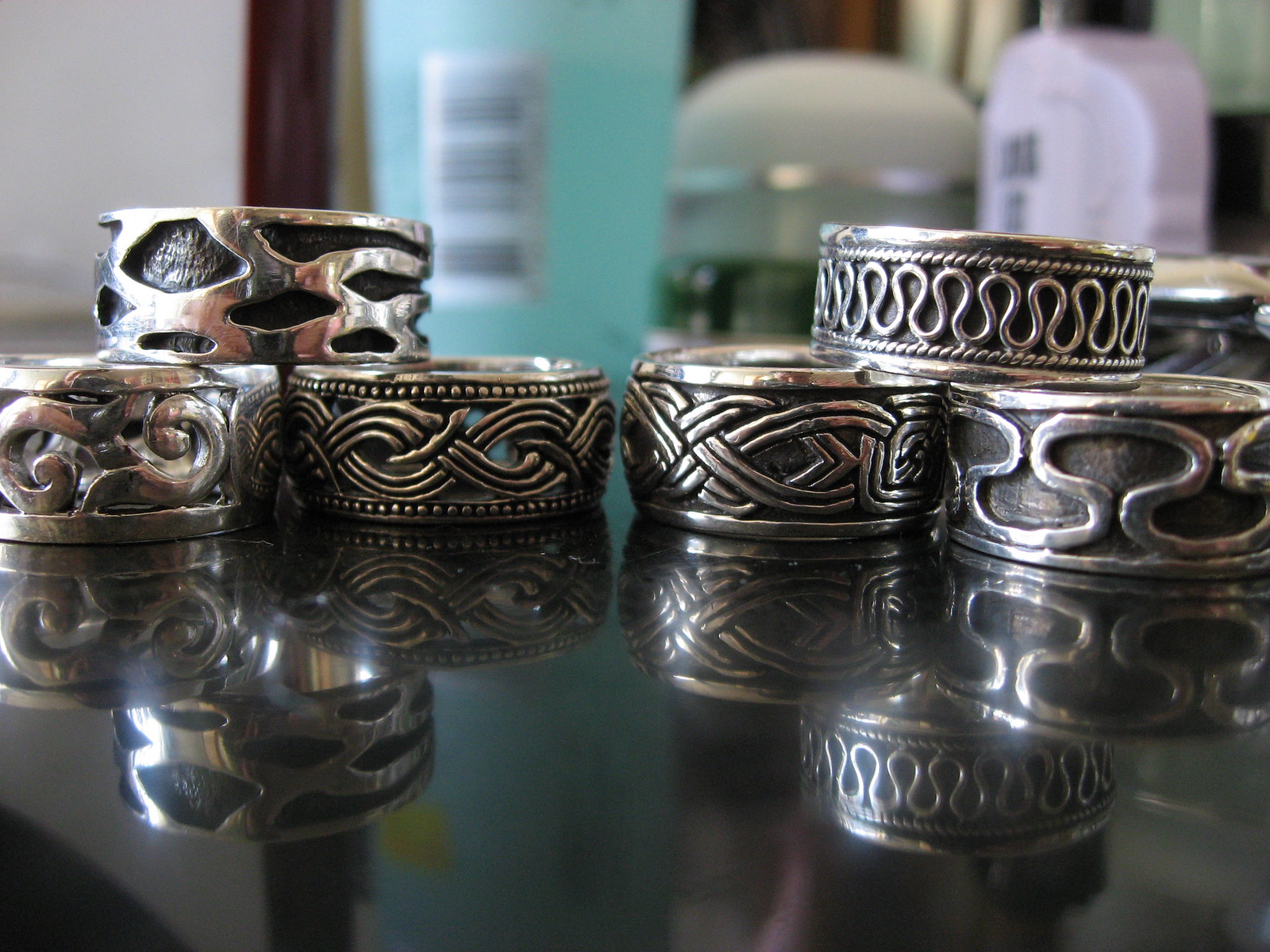This close-up color photograph captures an indoor scene featuring six silver finger rings with intricate designs, arrayed on a highly polished, reflective black marble surface. The rings are organized into two pyramidal stacks of three, with the top rings in each stack partially resting on the bottom rings. The rings exhibit ornate, raised patterns including braided, vine-like, and diagonal C-shaped lines, with variations of wave and accordion motifs. They appear to have a tarnished silver look, possibly by design. In the background, several out-of-focus bottles can be seen, containing various colored liquids—blue, pink, dark green, and white—adding a subtle depth to the composition.